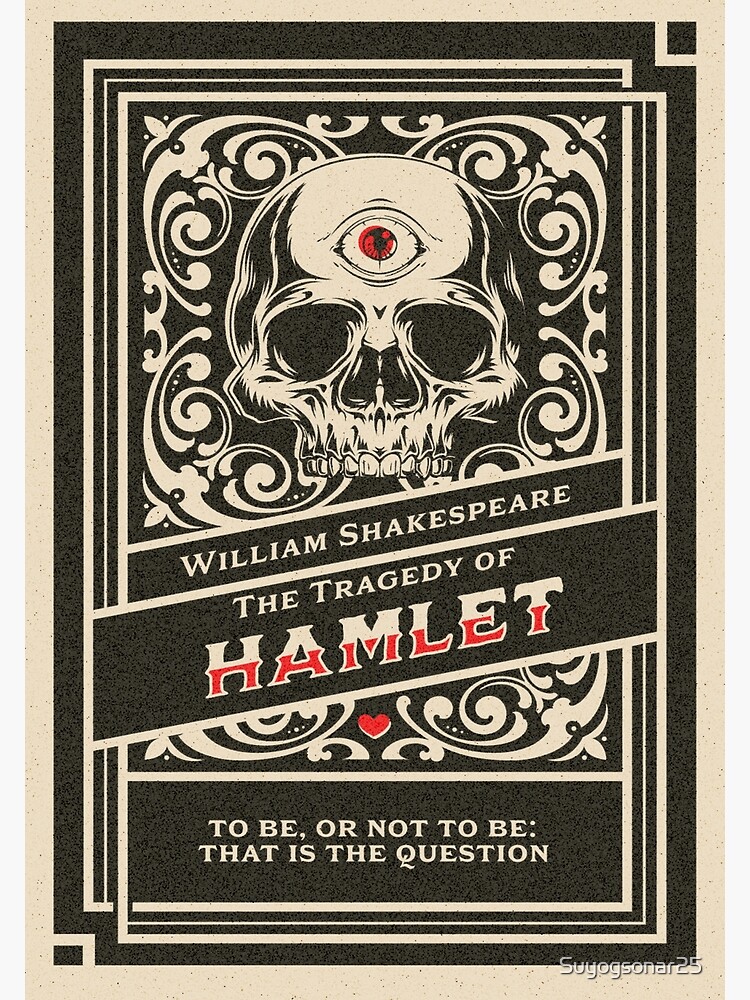The image is a stylized and reimagined digital poster for William Shakespeare's classic play, "Hamlet." Dominated by a black, white, and red color scheme, the poster features a central black-and-white skull with a red iris third eye, giving it a haunting and eerie feel. Intricate white filigree designs embellish the top half, enclosed within Art Deco style black borders. Below the skull, two slightly diagonal banners carry the text: the top black banner with white letters reading "William Shakespeare" and the larger bottom banner with white letters at the top stating "The Tragedy Of," followed by "Hamlet," where the letters transition from white at the top to red at the bottom. Further down, a small red heart is present, and a black rectangle at the base of the poster showcases the famous quote in white text, "To Be Or Not To Be, That Is The Question." Overall, the poster aims to present "Hamlet" with a modern, creepy twist.